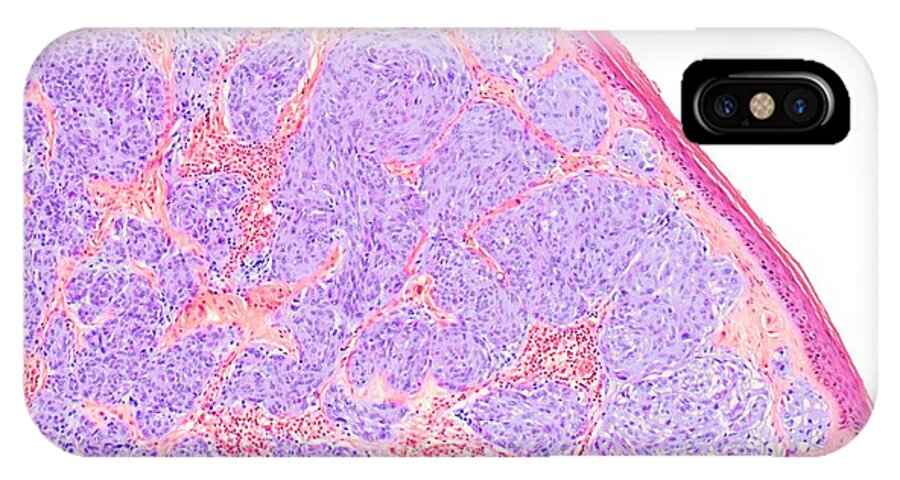This image showcases a brightly colored phone case, characterized by an intricate, swirly design that covers about 75% of its surface. The design features abstract patterns in shades of purple, pink, and red, reminiscent of a tie-dye effect or a photograph taken through a microscope. The remaining 25% of the case is a solid white area located towards the top right, which also includes a cut-out for the phone's camera. The phone case's overall texture and colorful patterns suggest a visually appealing but basic design, possibly for an older iPhone model or another smartphone, indicated by its curved edges and standard cut-out for the camera lens. This detailed and vibrant phone case seems like a standard, budget-friendly accessory that one might find in a store display or an advertisement.